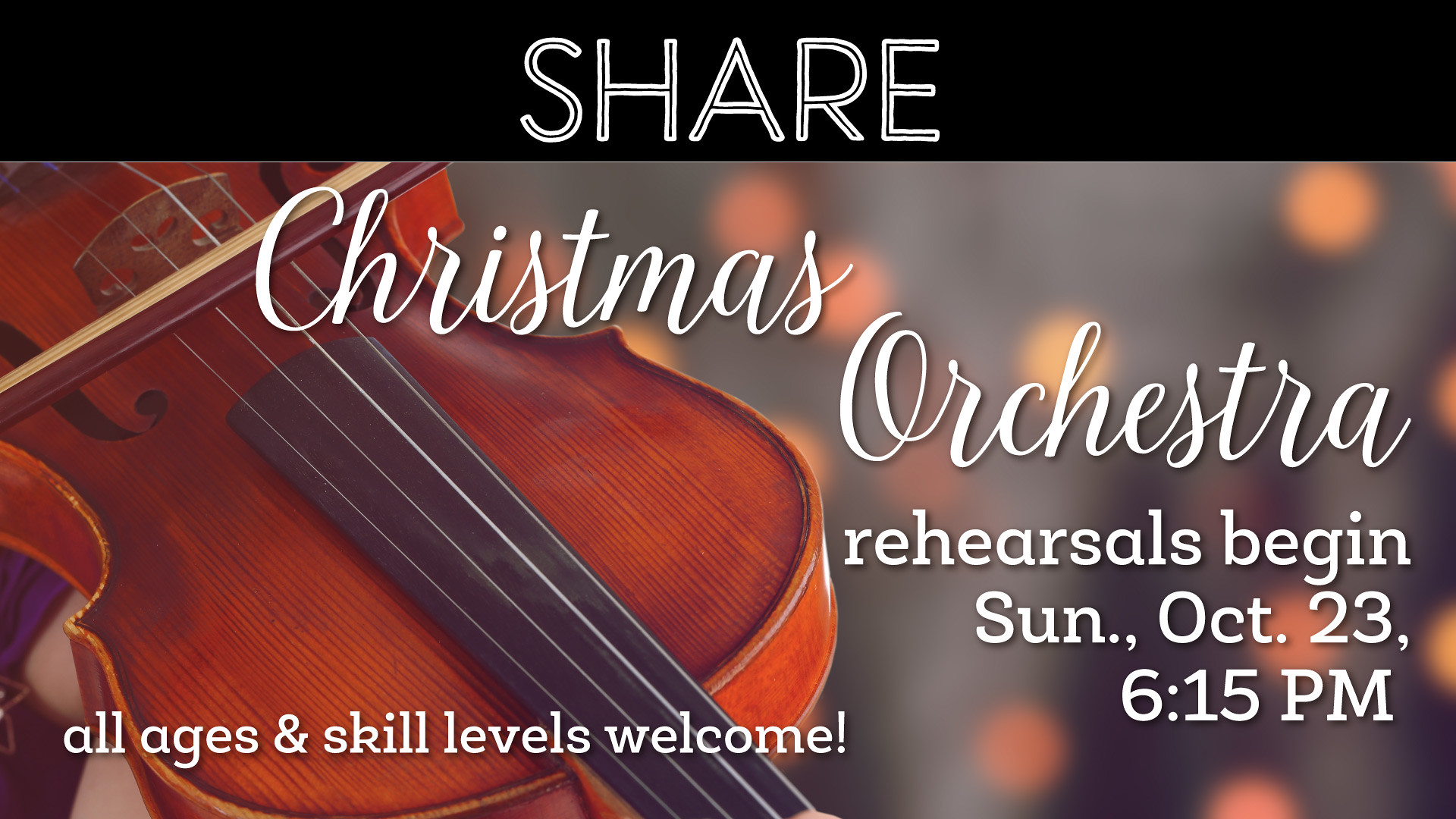This image appears to be an announcement card or advertisement for a Christmas orchestra. At the top, there is a thick black border with the word "SHARE" written in white, capital letters. Below this border is an illustration of a violin. The bottom of the violin is positioned at the top left corner of the image, with the handle extending downwards and off the image near the middle bottom. A bow is depicted across the strings at the upper left part of the violin. 

Across the top of the violin, it says "CHRISTMAS" in white lettering, and just below this, also in white, it says "ORCHESTRA." Beneath that, still in white print, it reads "REHEARSALS BEGIN," followed by "SUNDAY, OCTOBER 23," and "6:15 PM." Additionally, in the lower left corner, slightly overlapping the violin, the text "ALL AGES AND SKILL LEVELS WELCOME!" is written in white. The background to the right of the violin is blurry, featuring abstract shapes and dots in orange, yellow, and gray tones.